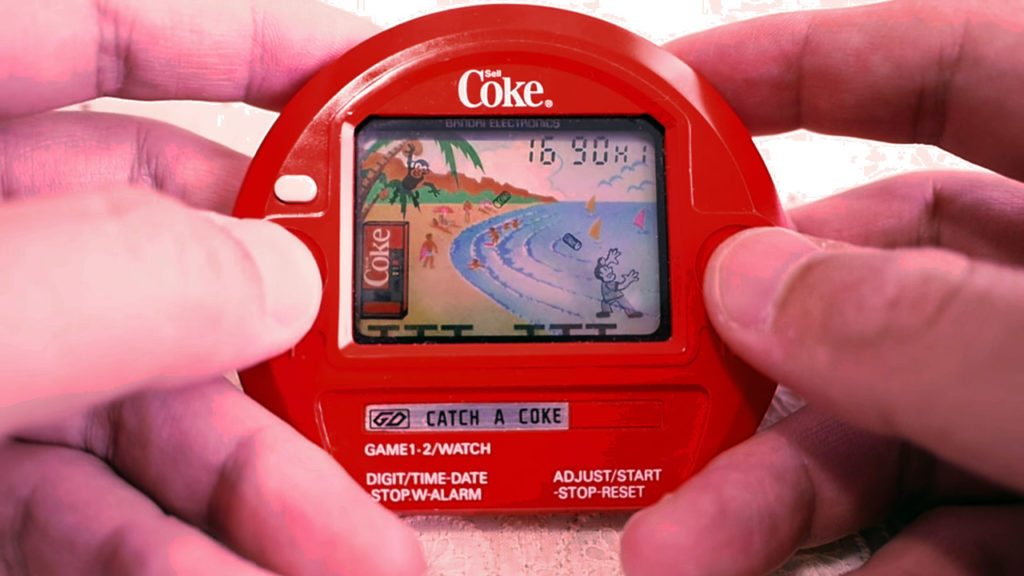In this color photograph, a person's hands are holding a small, red, handheld video game device against a white background. The device is semi-circular with a flat bottom. Prominently displayed at the top of the device is the word "Coke" in white letters, denoting the Coca-Cola brand. The central feature of the device is a small, color screen displaying a cartoon-style video game scene. The game screen depicts a beach setting with sand, palm trees, various human figures, and a Coke vending machine.

On the right side of the device, the person is pressing a button with their right thumb, while a white button is visible on the left side. Below the screen is a silver strip with the phrase "Catch a Coke" inscribed on it. Underneath this strip are several labels, including "Game 1-2/Watch", "Digit/Time-Date", "Stop W/Alarm", "Adjust/Start", and "Stop-Reset". The photograph captures the detailed interface and interactive elements, conveying the nostalgic charm of early handheld video games branded with Coca-Cola imagery.